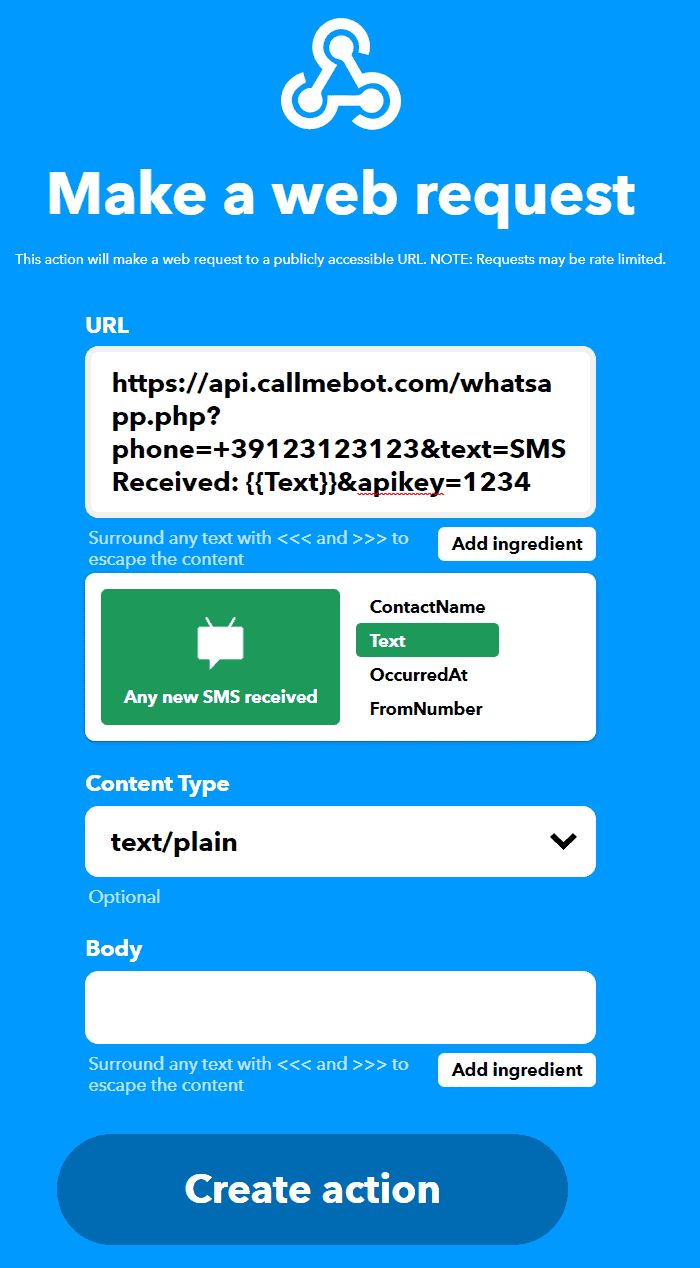A screenshot features a blue background with a distinct interface layout. At the top center, there is a prominent white symbol resembling an "A" with circular embellishments at the points of the letter. Directly below this symbol, large white text reads "Make a web request," capturing immediate attention. Beneath this, in thinner white font, a descriptive sentence informs users, "This action will make a web request to a publicly accessible URL. Note requests may be rate limited."

Further down, a white bar labeled "URL" is positioned above a text field containing an “HTTPS” web address, ready for the user to input or review. Below this URL entry, an instructional sentence in white text advises, "Surround any text with the less than sign and greater than sign to escape the content." To the right side of this instructional line, a button titled "Add ingredient" is visible, poised for user interaction.

At the bottom of the screenshot, there is a white box containing a green label which states, "Any new SMS received," signifying a specific condition or action related to incoming SMS messages. The overall design is minimalistic yet informative, guiding users through the process of making a web request with clear, concise instructions.